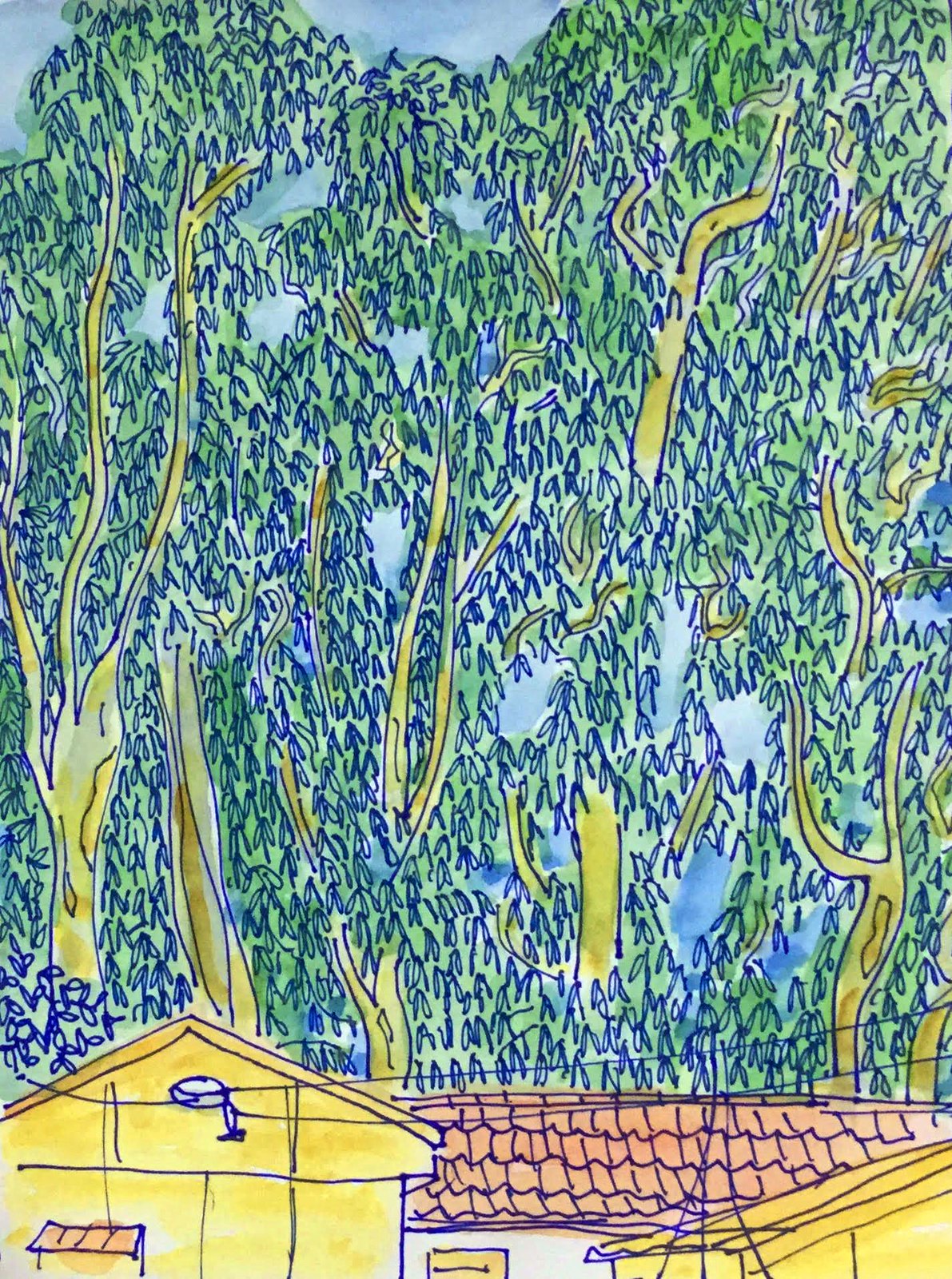This image features a child's drawing that resembles a whimsical watercolor painting. Dominating the bottom left of the artwork is a yellow house with a triangular, peaked roof made of brown, clay-like storm tiles. A silver or white light emanates from the center of the house's front. Power lines swoop from the left and stretch across the scene. Just visible on the left side is a doorway covered by a small red awning, and further to the right, you can spot the top of another house with a red roof and a white wall with a yellow door. Beyond these buildings, the top two-thirds of the image are filled with green trees with yellowish-brown branches, resembling tall weeping willows with spindly, droopy leaves. The blue sky is visible through the sparse foliage, adding a backdrop of color to the child's imaginative creation.